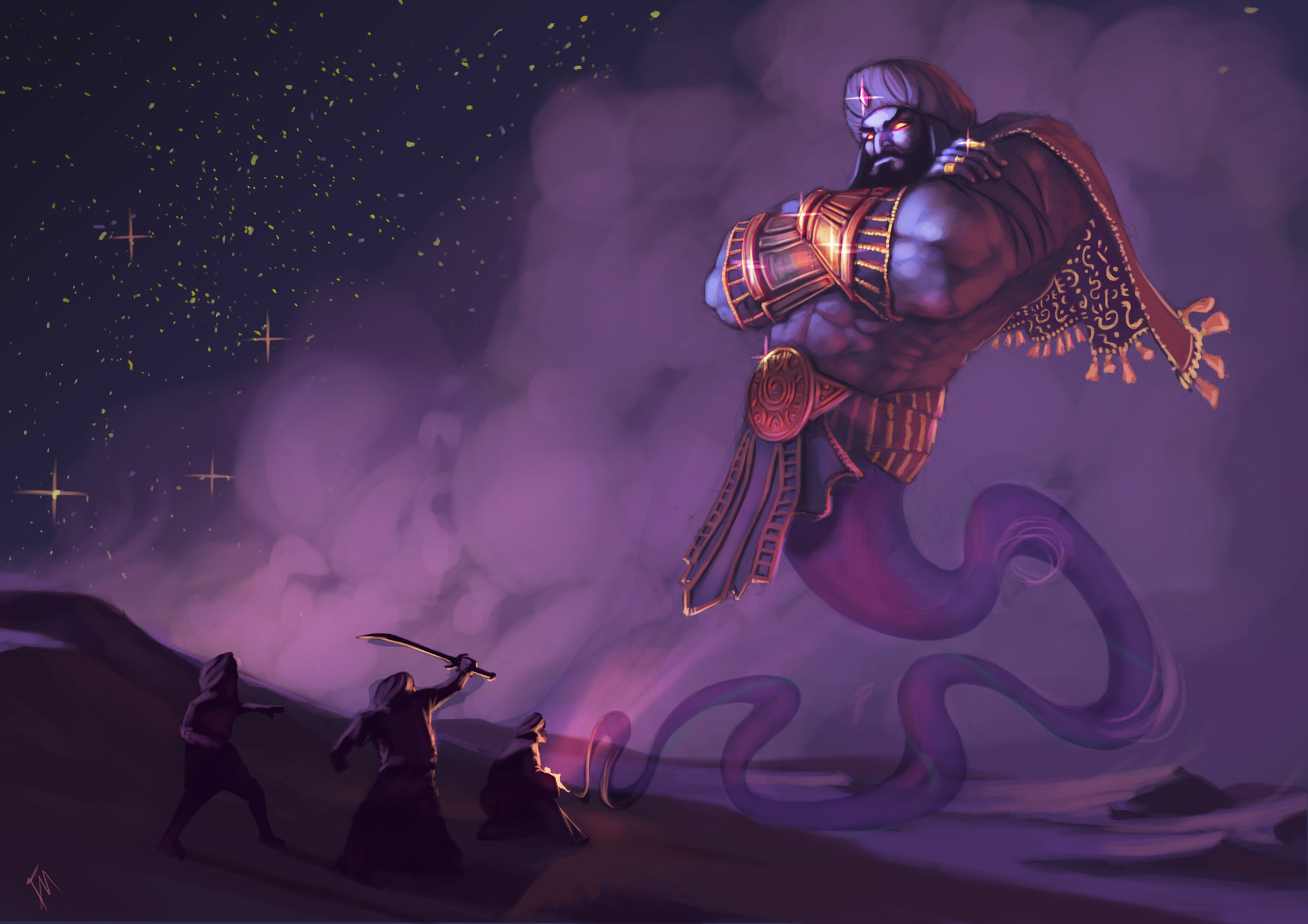The image is a vivid, nighttime fantasy illustration set at the ocean's edge, bathed in shades of dark purple and black. In the star-speckled sky, a massive, muscular genie with a black beard and glowing orange eyes emerges from a swirl of purple smoke. The genie, adorned in a jeweled turban, arm armor, a large belt, and a flowing cape, looms menacingly from the clouds.

On the beach below, three frightened men are captured in the bottom left corner. The man in the middle raises a sword toward the genie, while the man on the right clutches a lamp from which the genie has sprung. The third man stands back, appearing shocked. The landscape, lit under an eerie glow, is enveloped in purplish smoke, creating a dramatic and mystical scene.